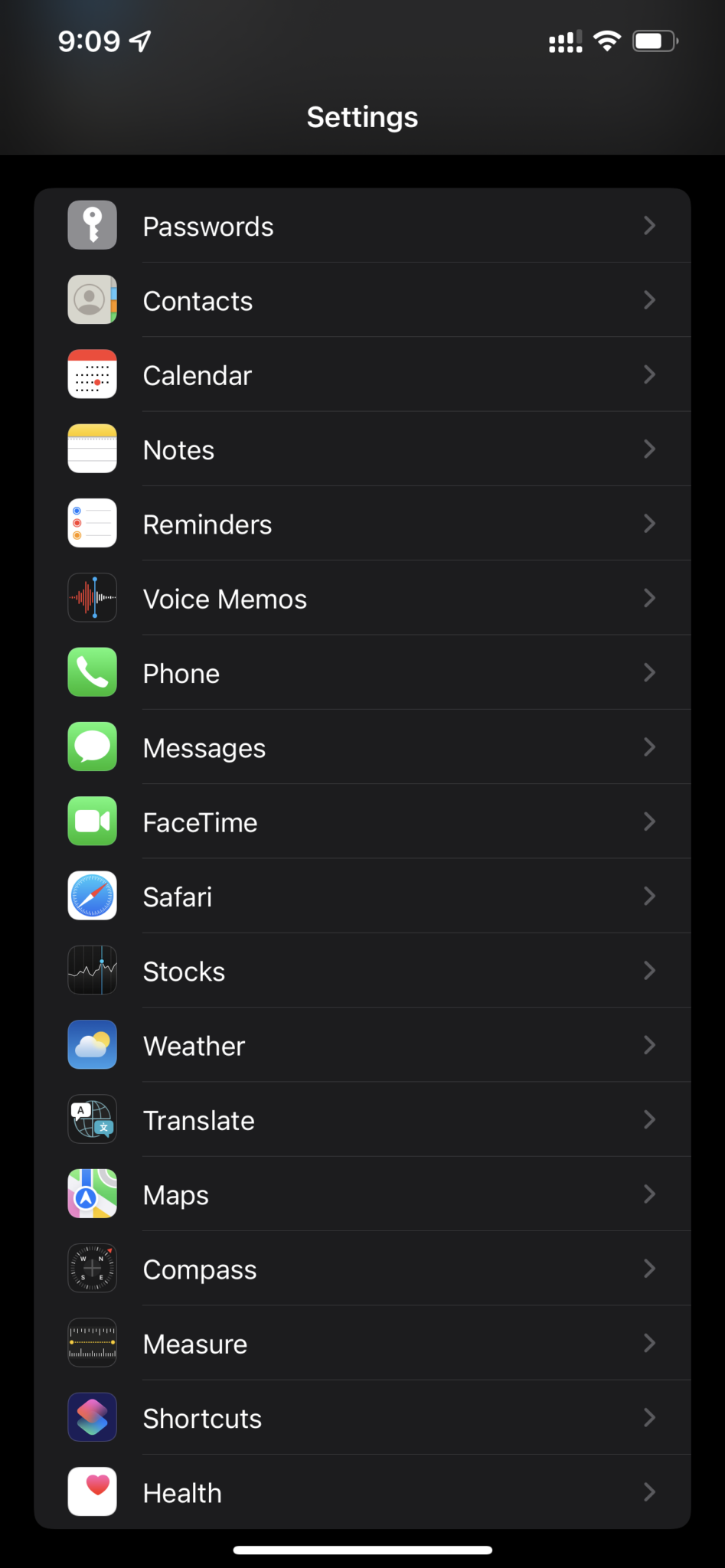The image depicts an iPhone with its settings page open. In the upper right-hand corner, the battery life is nearly full, and the device shows a strong cellular connection with almost all bars filled. The time displayed is 9:09. The settings page features a black background with the title "Settings" prominently displayed in white at the top center.

The screen lists several options with corresponding icons: Passwords, Contacts, Calendar, Notes, Reminders, Voice Memos, Phone, Messages, FaceTime, Safari, Stocks, Weather, Translate, Maps, Compass, Measure, Shortcuts, and Health. Each listed option has a small right-facing arrow to its right, indicating that tapping on any of these will lead to further submenus where users can adjust settings related to that specific category.